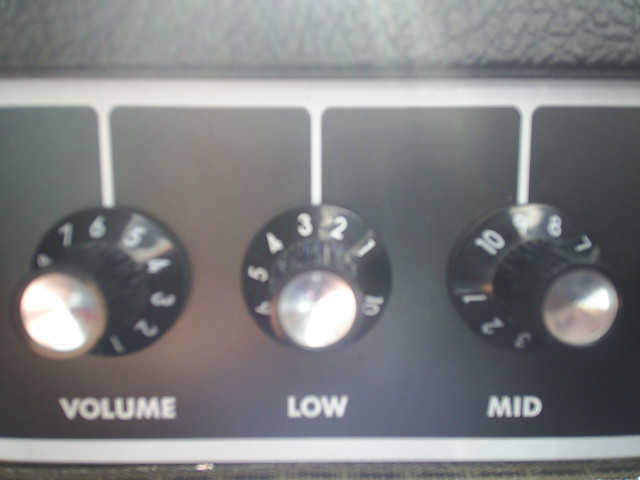This image is a blurry, close-up shot of what appears to be a section of a guitar amplifier control panel, possibly a Marshall amp. The central feature includes three black knobs with silver caps, designed with ridged sides for better finger grip and flared bases. Each knob is set against a black interface with white lines and numbers indicating their settings from 1 to 10.

The first knob on the left is labeled "VOLUME" in white letters and is currently set to six. The second knob in the center is labeled "LOW" or "LEVEL" (due to some discrepancy in the description) and is positioned at nearly three. The third knob on the right, labeled "MID," is almost dialed to nine. The overall panel is framed by a white outline, and above and below this control section, a faux leather surface, likely black, is visible, adding to the classic amplifier aesthetic. The background of the image is gray and blurry, highlighting the detailed yet low-quality close-up of the amp controls.